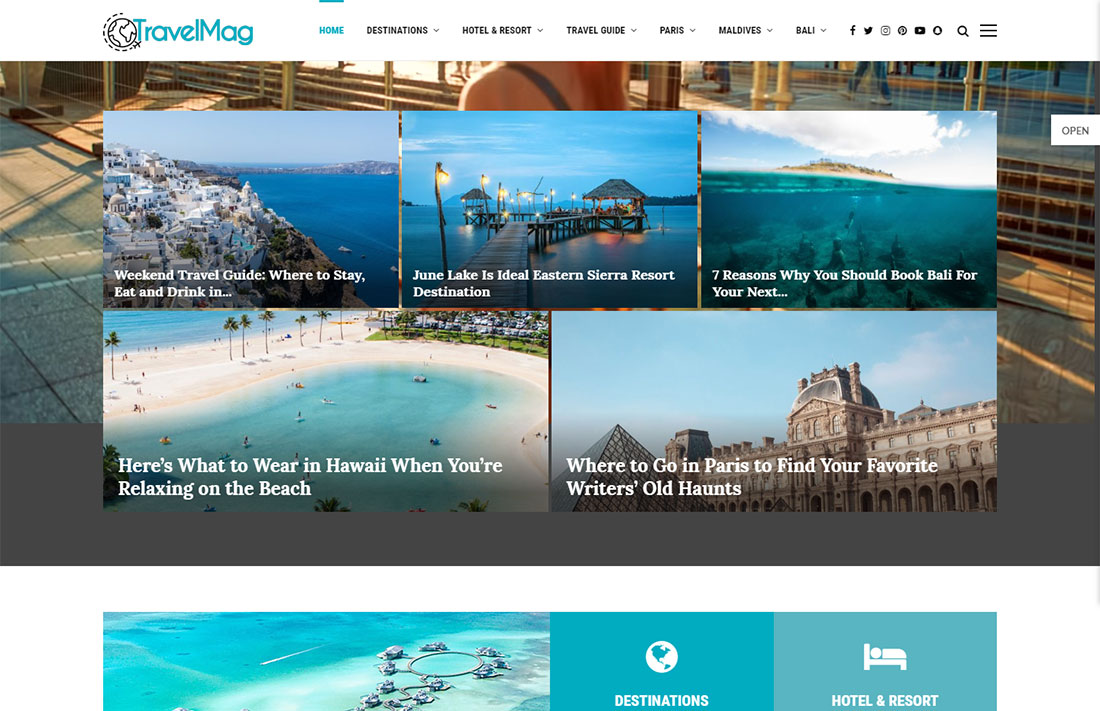This image showcases the TravelMag website, which is a hub of picturesque travel destinations photographed in stunning daylight. The homepage, highlighted in blue, features a range of sections such as "Home Destinations," "Hotel and Resort," "Travel Guide," along with popular destinations like Paris, the Maldives, and Bali. The vibrant visuals include serene waters and scenic outdoor settings. The website also offers social media links, including Facebook, Twitter, Instagram, and Pinterest, for wider connectivity.

A search bar icon represented by a magnifying glass allows users to explore specific travel content. A highlighted section, "Weekend Travel Guide: Where to Stay, Eat, and Drink," presents a captivating view of a foreign city by the ocean. Another feature showcases June Lake as an ideal evening destination in the Eastern Sierra, complete with tiki huts and a lighted wooden bridge over water.

There is also a compelling post titled "Seven Reasons Why You Should Book Bali for Your Next Trip," featuring clear waters and a backdrop island against a pristine sky. Another section, "What to Wear in Hawaii When Relaxing on the Beach," displays a Hawaiian beach scene with people enjoying the water and diverse sands at a resort. For literature enthusiasts, the site advises "Where to Go in Paris to Find Your Favorite Writers' Haunts," accompanied by an image of a historic Parisian building.

The bottom of the webpage includes navigation options labeled "Destination," "Hotel," and "Resort," offering an extensive range of choices for planning the perfect trip.